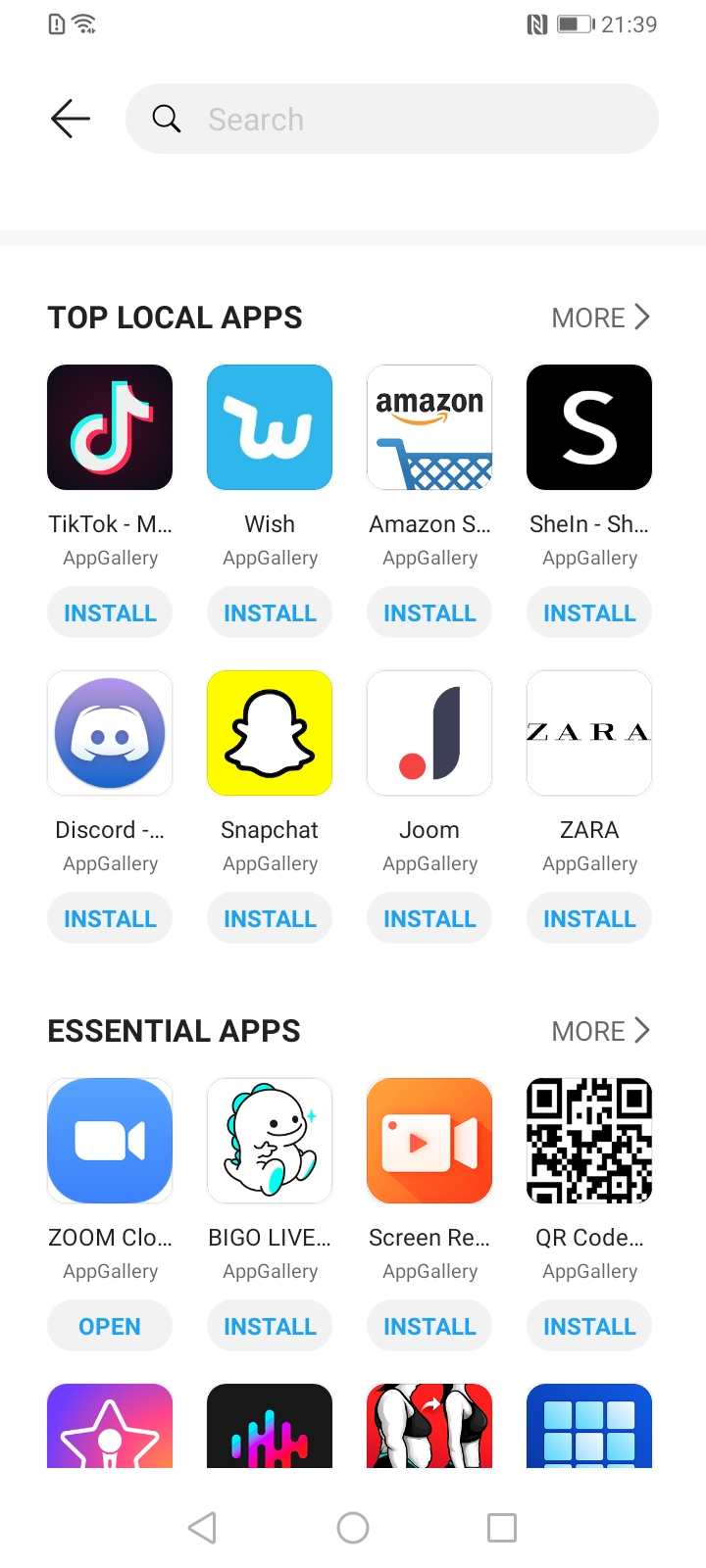The image depicts a smartphone screen displaying a selection of apps available for download. At the top, there's a grey back arrow and a search function, with the section titled "Top Local Apps." The listed apps include TikTok, Wish, Amazon, Shein, Discord, Snapchat, Zoom, and Zara, each accompanied by their respective icons. 

Below this, there's a category labeled "Essential Apps", featuring apps such as Zoom, BIGO LIVE, a QR code scanner, and another app whose name isn’t fully visible. Most apps are displayed with identifiable icons and names corresponding to their services. 

The background is predominantly white, with black text and colorful app logos. Blue "Install" buttons are present next to the majority of the apps, while the Zoom app shows an "Open" button, indicating it is already installed on the device. 

At the very bottom of the screen, standard navigation buttons are visible: a back button, a home button represented by a circle, and a recent apps button depicted by a square. The top status bar of the screen shows icons for Wi-Fi, battery percentage, and the current time, underscoring that the image likely represents a view from an app store interface.